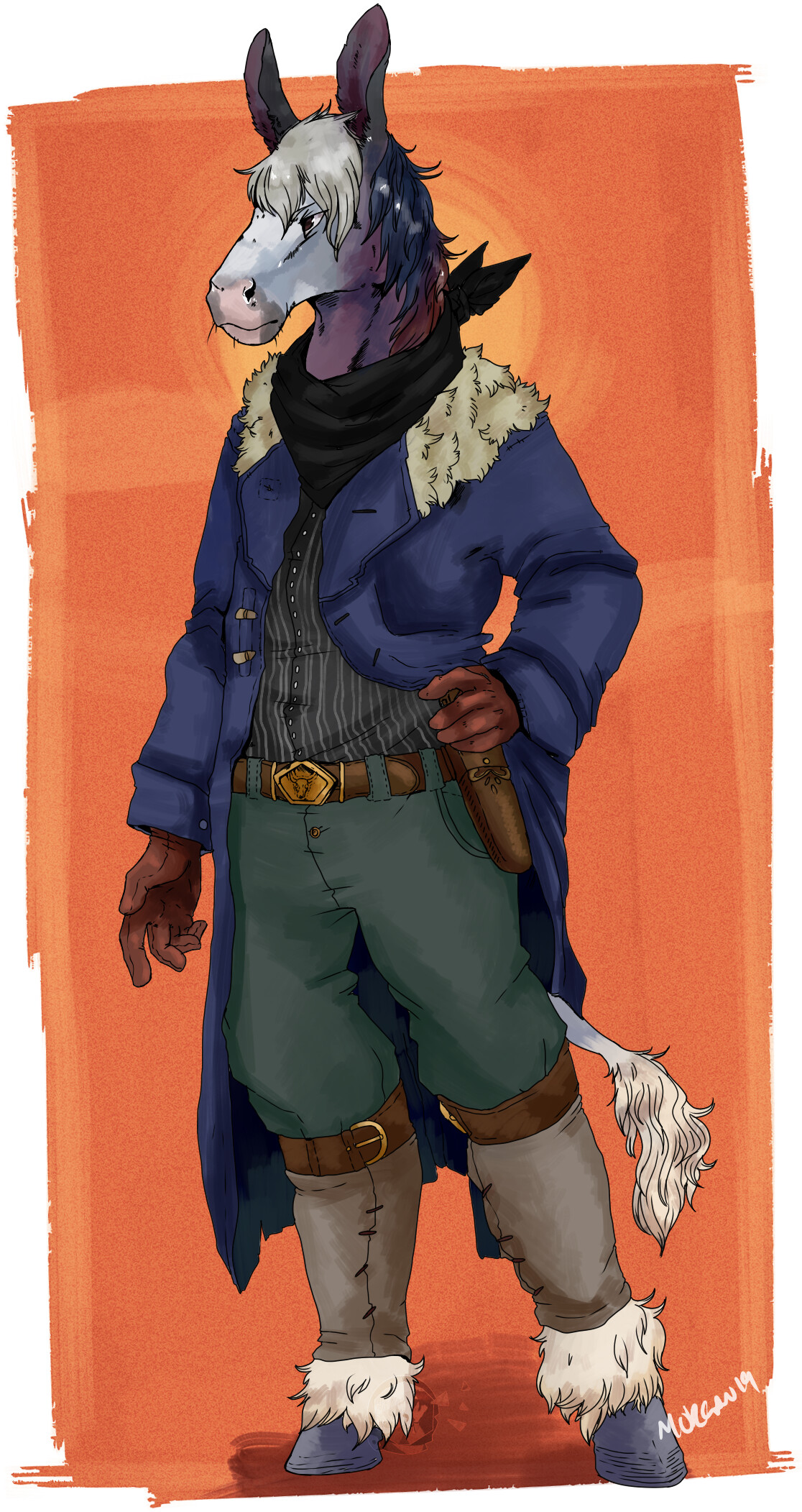The painting features a fantastical, anthropomorphic character, which could serve as a concept for a comic book, movie, or other media. This character has the body of an upright horse or similar creature. It stands against a vibrant orange background, with hues of light and dark oranges, and a round, lighter orange element resembling the sun behind it.

The character has a horse-like face, grayish-blue in color, with a darker gray forelock. The ears are straight and reminiscent of a horse, darker in shade. It features purple hues transitioning into the body, crowned with white or blonde hair on top of its head. The character is adorned in a blue jacket with a fur collar and is also wearing a black bandana tied around its neck.

Dressed in green pants with a brown belt, the character also sports brown leather gloves over its hands. Its feet end in hooves surrounded by fur, and a cow's tail sticks out from the side of the jacket. Completing its outfit are boots with buckles at the top. The character stands upright, with one hand on its hip, exuding a sense of readiness and confidence.